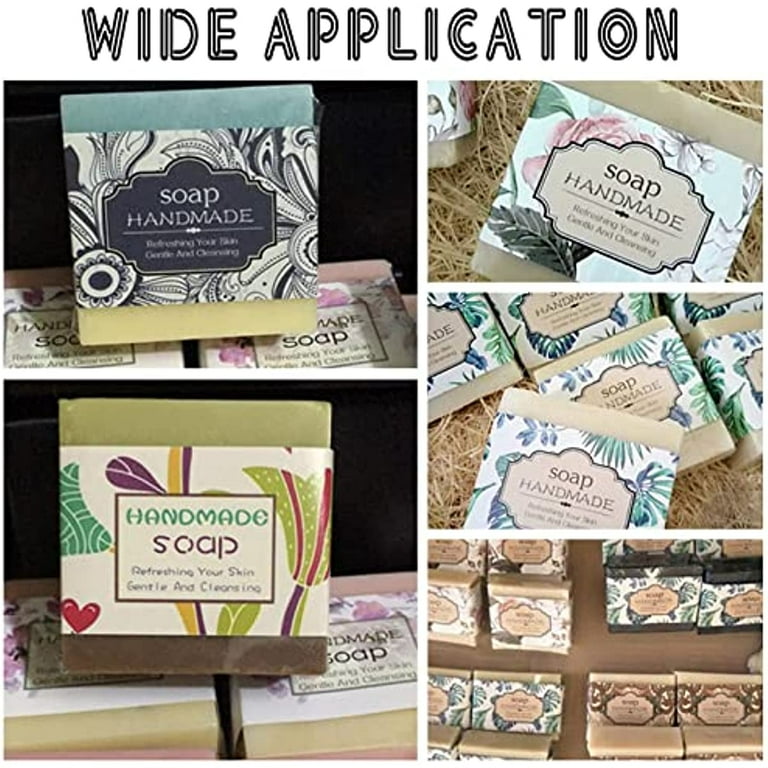The image is a collage featuring an assortment of handmade soaps showcased as a potential advertisement. The title, written in a somewhat hard-to-read black font, prominently reads "WIDE APPLICATION." Below the title are five smaller photographs arranged in two columns. The top left image features a blue and yellow bar of soap standing upright on two flat-lying soaps, labeled "SOAP HANDMADE." Below it, the soap is tan and dark brown, covered in a colorful label with shades of olive green, red, and purple, and the text "HANDMADE SOAP GENTLE AND CLEANSING REFRESHING YOUR SKIN."

Moving to the right column, the top two images each show a single-toned tan soap. The one in the upper right has a decorative, vintage-looking floral wrap that says "SOAP HANDMADE," and it is presented on a bed of hay. The middle right image is another tan soap, similarly wrapped. The bottom right image showcases a variety of small soap bars arranged in neat rows, with hints of green tea and chocolate colors, suggesting different ingredients and scents. The overall aesthetic is rustic and homemade, enhanced by the seemingly unprofessional graphic design.